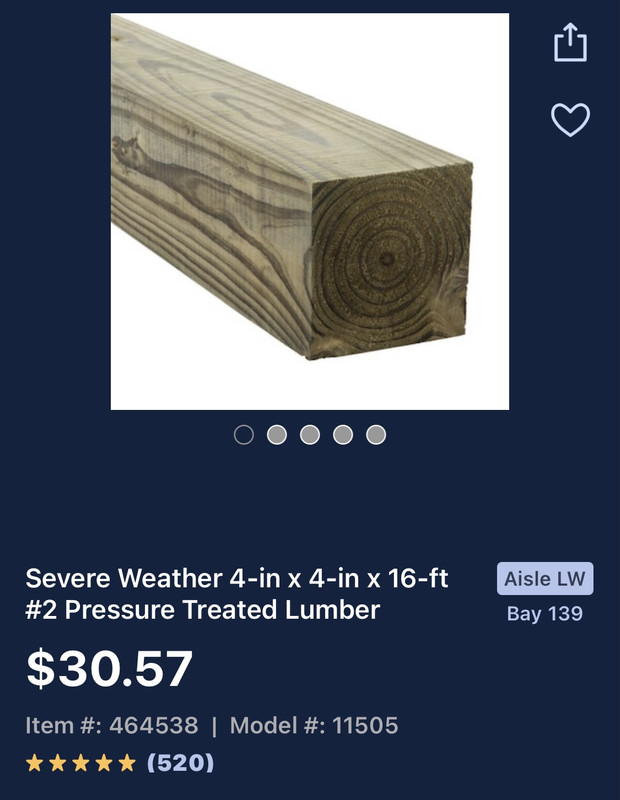The image features a dark blue background with a forward button in the top right corner and a heart icon slightly to the left of it. To the left of these icons, there is a prominent white square that showcases a central piece of lumber. This piece of lumber appears to be a 4x4, cut into a cube shape, prominently displaying its bottom face and two adjacent sides. The face directed towards the camera exhibits a distinctive round tree ring. Below the white square is a gray-outlined circle centered in the image, surrounded by four smaller gray circles to its right.

Further down, white text provides detailed information about the lumber: "Severe Weather 4 in. x 4 in. x 16 ft. #2 Pressure-Treated Lumber $30.57. Item Number: 46 4538. Model Number: 11505." This text is accompanied by a five-star rating, based on 520 reviews, indicated within parentheses. Additionally, a light blue box on the right displays the text "I’ll W," with "Bay 139" written below it.